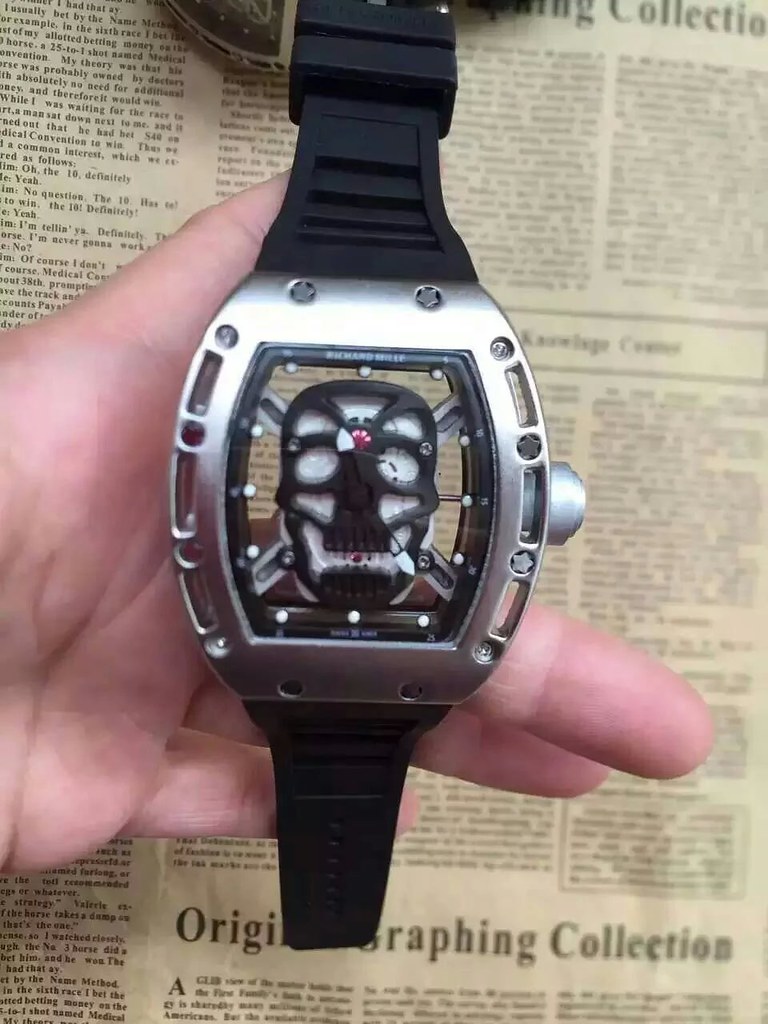The image features a watch face adorned with an intricate skeleton design in the center. The watch lacks visible mechanical parts but maintains the distinctive appearance of a timepiece. The face of the watch is predominantly black and white, with silver edging that adds a touch of elegance. A striking pink shell-like pattern embellishes the skeleton's forehead, and a small pink gem is nestled within the skeleton's teeth, adding a pop of color and a unique focal point.

The watch is held delicately by a hand, and the background consists of a newspaper with visible text. The lower part of the newspaper prominently displays the words "Original Graphing Collection." Another article on the newspaper mentions something about a "collection" and a "knowledge center," providing a textured backdrop that contrasts with the refined watch face.